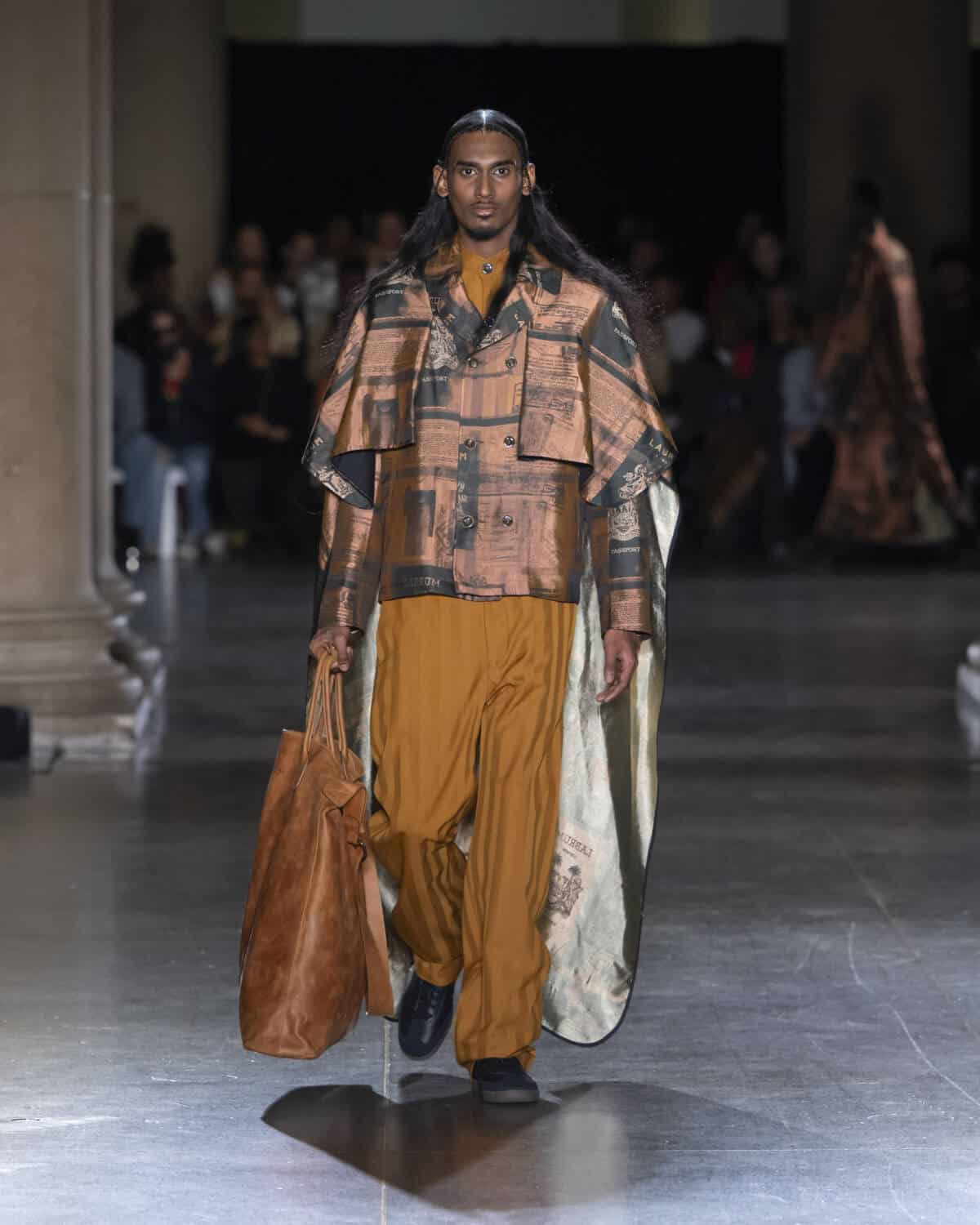The photograph captures a striking and fashionable man with a confident stride, as though he is on a runway. He has long, straight, dark hair that flows past his shoulders and is slicked back at the top. He is adorned in a loose-fitting, black and copper-patterned shirt with long sleeves, paired with baggy yellow pants. His sleek, stylish outfit is complemented by black shoes. Carrying a large, brown leather bag that nearly reaches the floor, the man commands attention. The setting appears to be indoors, featuring a gray, metallic-looking floor with white pillars to the left and a crowd of blurred, fashionably attired individuals in the background. The overall scene suggests a high-end fashion show, with the model firmly in focus against a dynamic yet atmospheric backdrop.